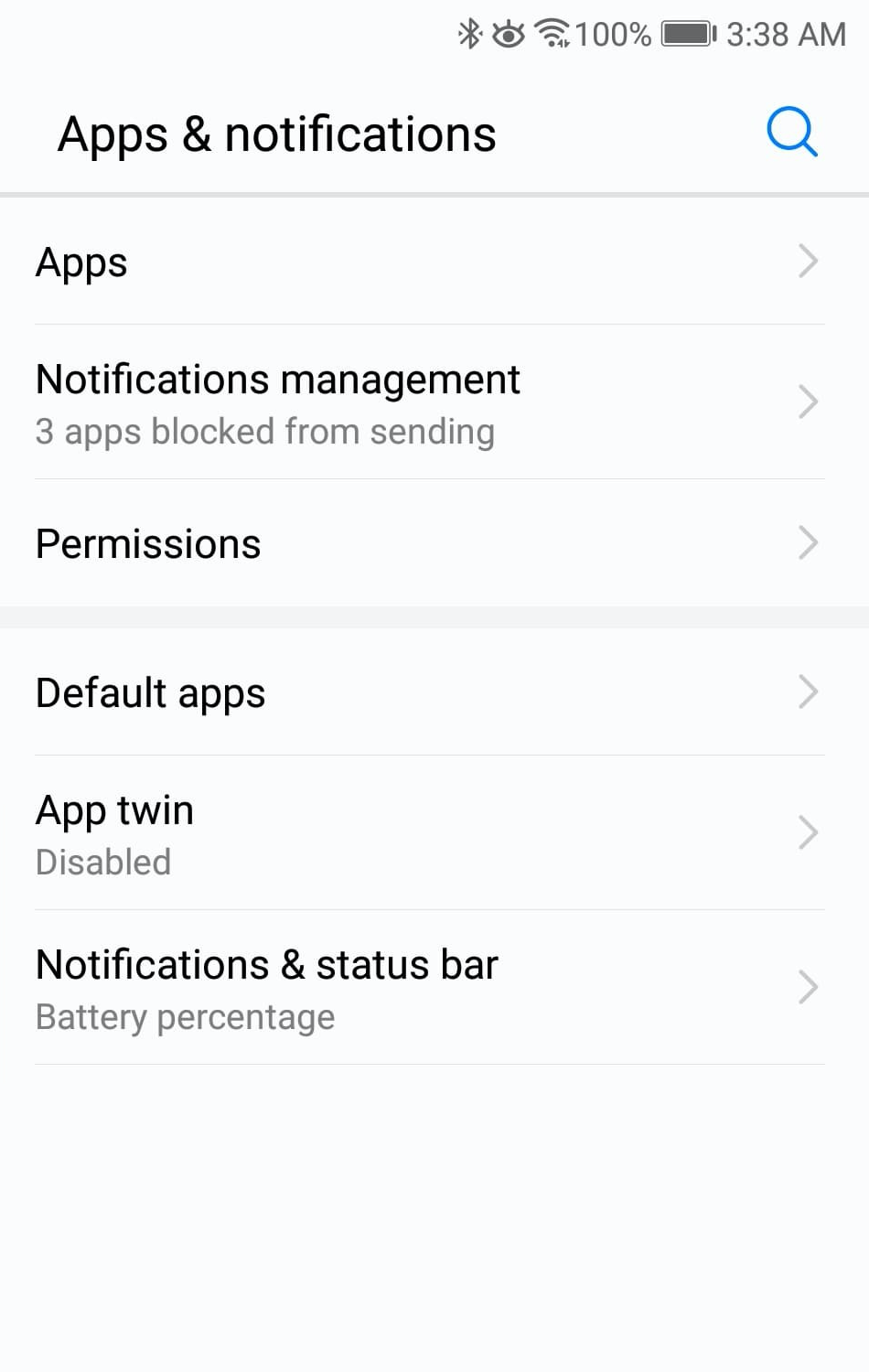This is a detailed screenshot of a phone's settings menu, displaying in sharp clarity with no pixelation or blurring. The top section of the image features a gray background with various status icons including a Bluetooth symbol, a stylized eye with visible pupil and eyelashes, a Wi-Fi signal that slightly resembles a funnel or tornado, and a battery icon showing 100% charge. The time displayed is 3:38 a.m.

Below this header, the settings options are organized in a white background with black and gray text. The topmost option is labeled "Apps & notifications," adjacent to a blue magnifying glass icon on the right. A thin gray line separates this header from the settings categories list, each accompanied by a pull-down arrow on the right.

The categories listed include:
1. Apps
2. Notifications Management - indicating "3 apps blocked from sending"
3. Permissions
4. Default Apps
5. App Twin - noted as "disabled"
6. Notifications & Status Bar - with a mention of "battery percentage"

The layout of the text is bold, user-friendly, and easy to read. The image exudes clarity, simplicity, and is devoid of any additional images or distractions.